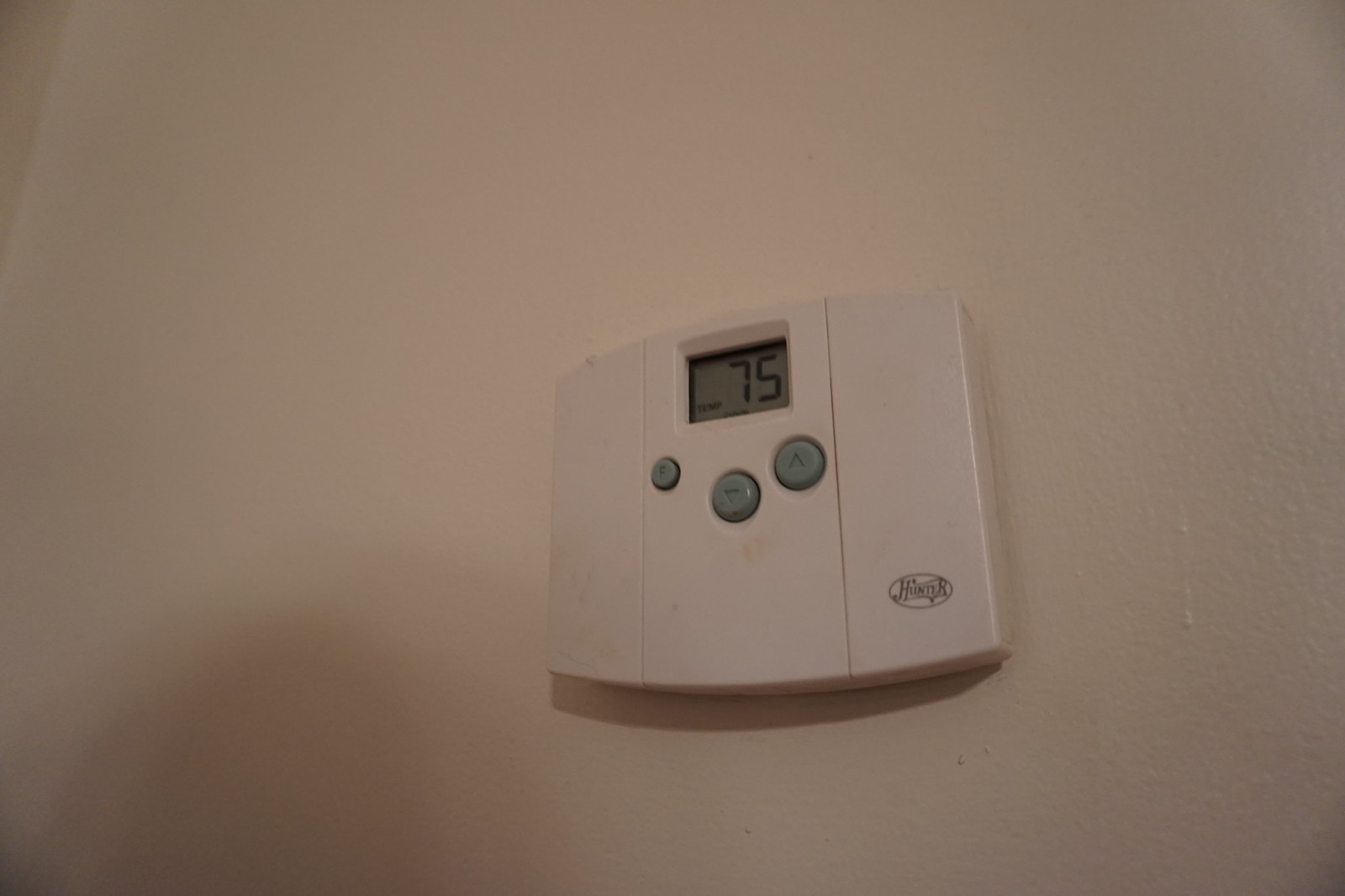This photograph captures a thermostat mounted on an ecru-colored wall with an eggshell finish, which features slight imperfections and small paint drips. The thermostat itself is an elegant white device with a unique parallelogram shape, characterized by bulging, rounded edges at the top and bottom. It sports a small door indicated by two vertical lines, suggesting that the front panel can be opened. At the bottom right, the thermostat features a sophisticated, brown, stylized logo that reads "Hunter."

The device is equipped with three gray buttons—an up arrow, a down arrow, and a smaller button marked with the letter "F." Prominently, there's a digital display window reading "TEMP" with the numerals "75" beneath it. Although partially obscured, additional text below the number likely indicates the system’s mode, possibly stating whether it is set to heat or cool. The digital nature of the unit suggests that more settings can be accessed, possibly scrolling through various functions. This leaves some ambiguity about whether the unit controls only heating or both heating and cooling systems.